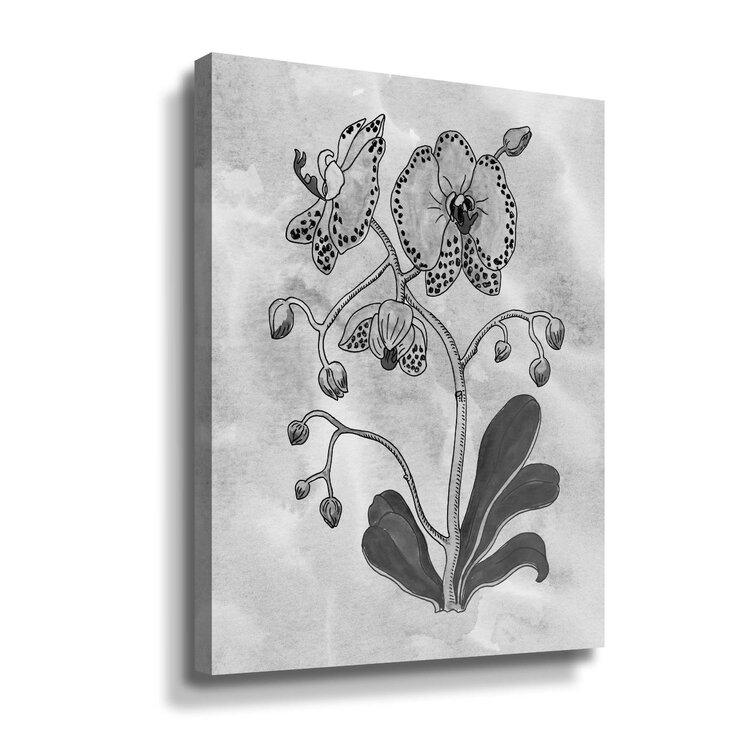Displayed prominently on a white wall, a black and white canvas picture captures the eye with its modern contemporary depiction of a flower. The stark contrast is striking due to the image being a monochromatic sketch. Protruding slightly from the wall, the canvas casts a soft shadow, emphasizing its dimension and placement. The flower, rendered in meticulous detail, starts from the bottom with darker leaves that possess rounded edges. As the eye travels upward along the main stem, it notices several buds yet to bloom, contrasted against three fully opened flowers. Each bloom is intricately drawn, showcasing solid petals adorned with black dots along the edges and inside. Additional smaller stems split off, bearing more unopened buds, adding to the layered complexity of the piece. A subtle detail possibly includes the initials of the artist etched onto the main stem. The overall impression is that of a finely crafted piece, perhaps done by an amateur artist, yet it evokes a simple elegance through its intricate line work and thoughtful composition.